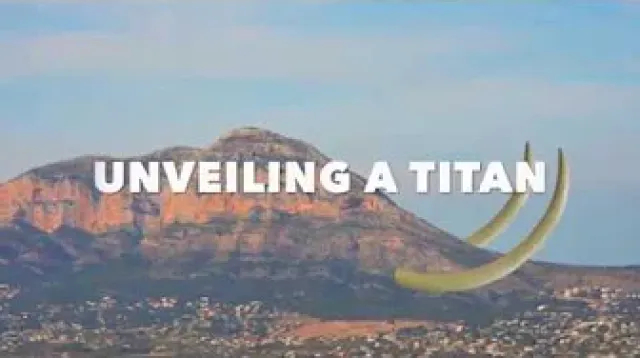The image depicts an expansive mountain range under a blue sky dotted with white clouds, set in what appears to be a western American desert. The scene captures the warm hues of either a setting or rising sun, casting a hazy light over the rugged landscape. Dominating the middle ground is a brown mountain, distinctive due to two large, upward-pointing tusks jutting out from its base, resembling those of a woolly mammoth. These tusks are an off-white, almost egg-white color, and their peculiar addition to the mountain suggests a playful, possibly mythological theme. In the very center of the image, thick, blocky white letters spell out "UNVEILING A TITAN," hinting at a mythical or adventure theme, perhaps for a show or movie. Below the mountain, the foreground features flat desert terrain, with the faint outline of a village or city, indicated by several small structures. The image's out-of-focus quality lends it a dreamlike ambiance, enhancing its otherworldly touch.